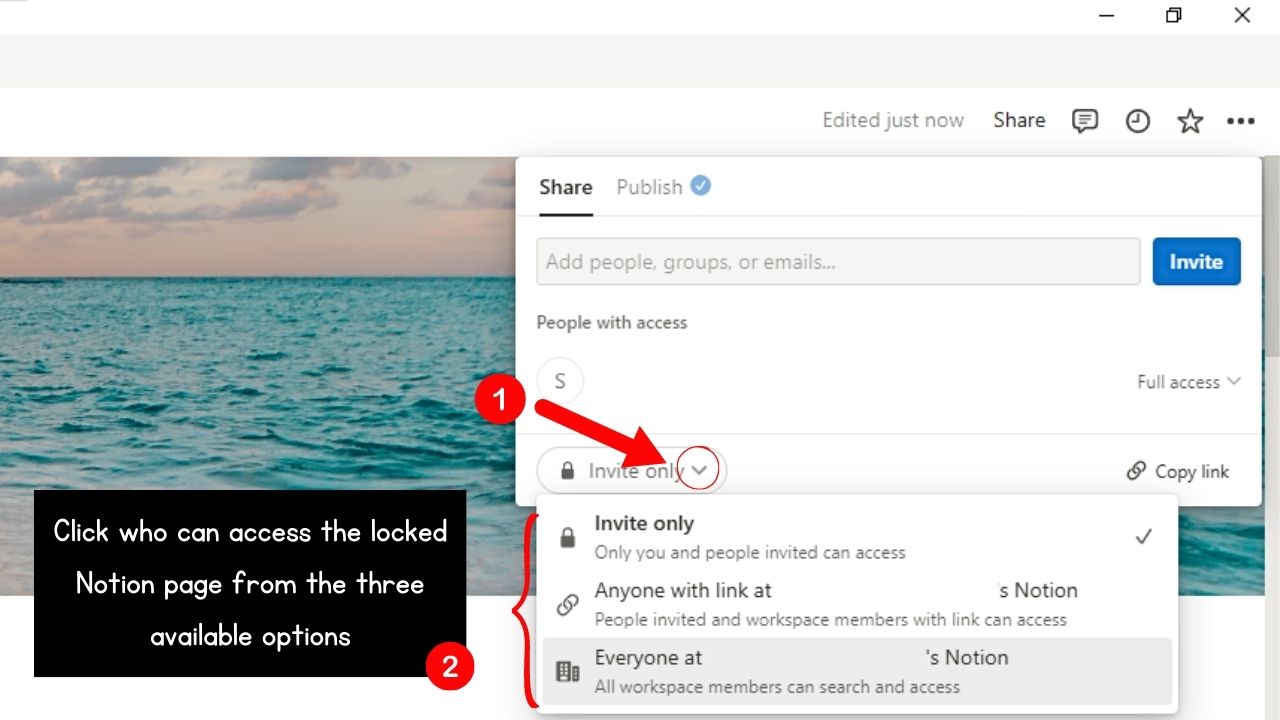A screenshot of an interface is shown, likely from a web-based application, featuring multiple UI elements and task options. In the top right corner, there are the standard window control icons: minimize, maximize, and close (X). Directly below these controls, an empty gray rectangle is visible. Below this rectangle, there is a label that reads "edited just now," and beside it, an option to "share." Next to a comment box, there are three icons: a clock, a star, and an ellipsis (…).

On the left side of the screenshot, there is an image depicting an ocean with a purple sky. Below this image is a black rectangle with white text inside, saying, "Click who can access the Locke Notion page from the three available options." In the bottom right corner of this black rectangle, there is a red circle with the number two inside it.

To the right of this rectangle, a white rectangular box contains the text "Share" and "Publish," accompanied by a blue circle with a check mark. Below this, a text box prompts the user to "add people, groups, or email," alongside a blue button labeled "Invite." Further down, a section titled "People with access" is visible, featuring a circle with an "S" inside it.

There is a drop-down menu labeled "Invite only," marked with a lock icon and an arrow pointing downward. Adjacent to this drop-down menu is a red arrow pointing at the downward arrow, with a circle containing the number one next to it.